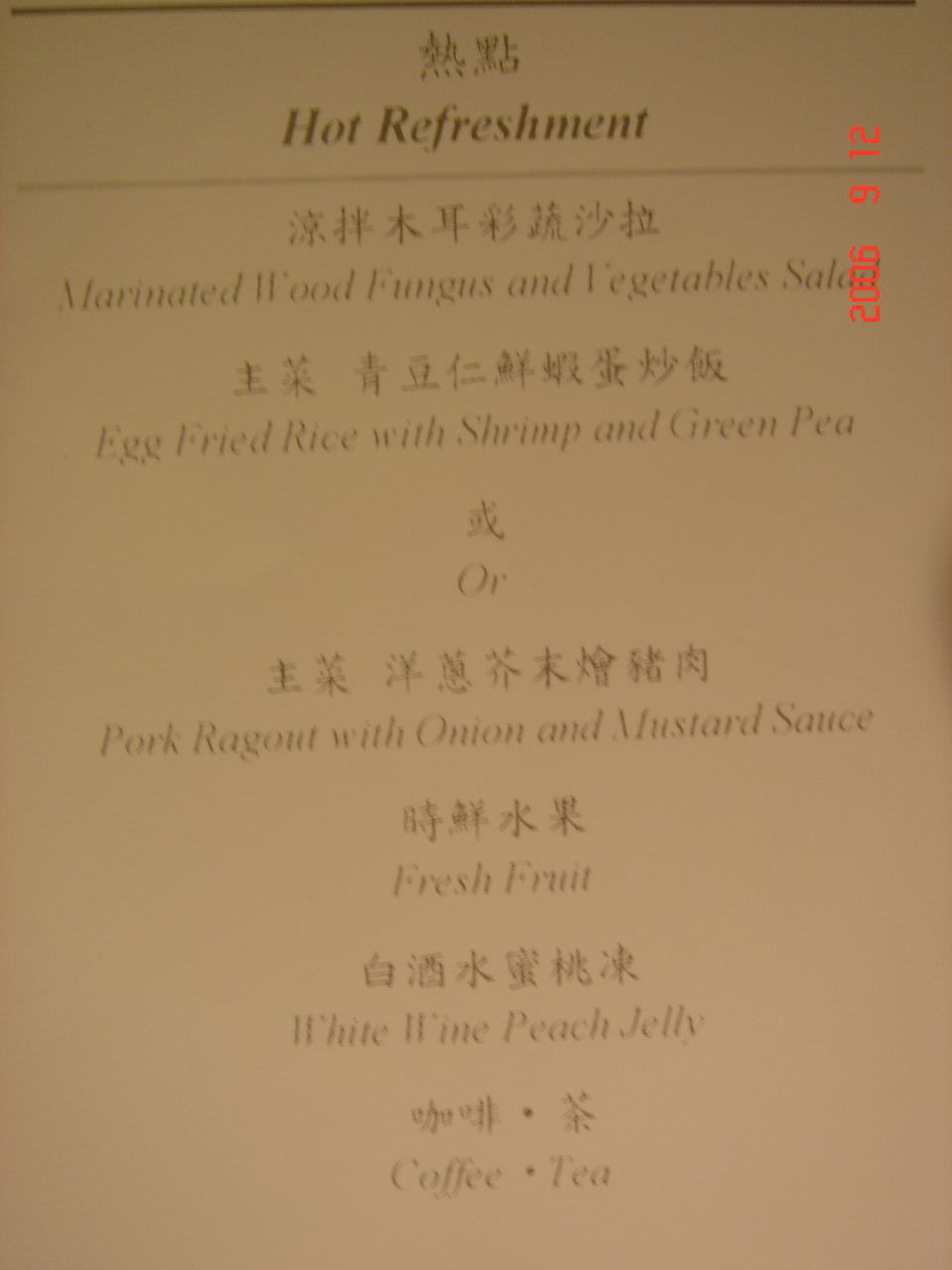In this image, you can see a menu printed on a sheet of paper featuring bilingual text in both an East Asian language—possibly Chinese—and English. The menu items are listed with their original foreign language text at the top and their English translations directly below. Specifically, the menu includes items such as "Hot Refreshments" and "Marinated Wood Fungus and Vegetable Salad" in both languages. Additionally, it lists various dishes including "Egg Fried Rice," "Shrimp and Green Pea," "Pork Ragout with Onion and Mustard Sauce," "Fresh Fruit," "White Wine," "Peach Jelly," and options for "Coffee" and "Tea."

To the right side of the paper, there is a numeral figure "2006" and a specific date, "September 12th," marked in red, possibly indicating when the menu was last updated or the photograph was taken. The main text of the menu is in a light gray color. This detailed image appears to be of a bilingual food menu with its textual content carefully delineated, allowing readers to discern and compare the menu offerings in two distinct languages.